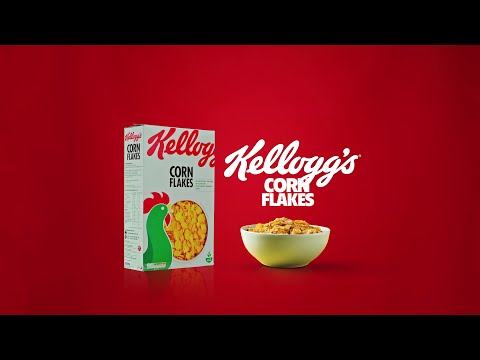In this advertisement for Kellogg's Corn Flakes, a box of the cereal is prominently displayed against a vivid red background, bordered by thick black horizontal bars at the top and bottom. The white cereal box features the iconic red Kellogg's logo at the top, though the second "G" and the apostrophe "S" are slightly cut off, suggesting they wrap around the box. Below the logo, "Corn Flakes" is printed in black. The front of the box showcases a green rooster with a red comb and wattles, accompanied by an overhead view of a bowl filled with Corn Flakes. To the right of the box, the words "Kellogg's Corn Flakes" are written again in white with the cursive "Kellogg's" logo, followed by "Corn Flakes" in black. Below this text, a white bowl, casting a delicate shadow, brims with a generous serving of the cereal. The bowl, filled nearly to a third of the box's height, emphasizes the plentiful serving size, all set against the consistent red backdrop.